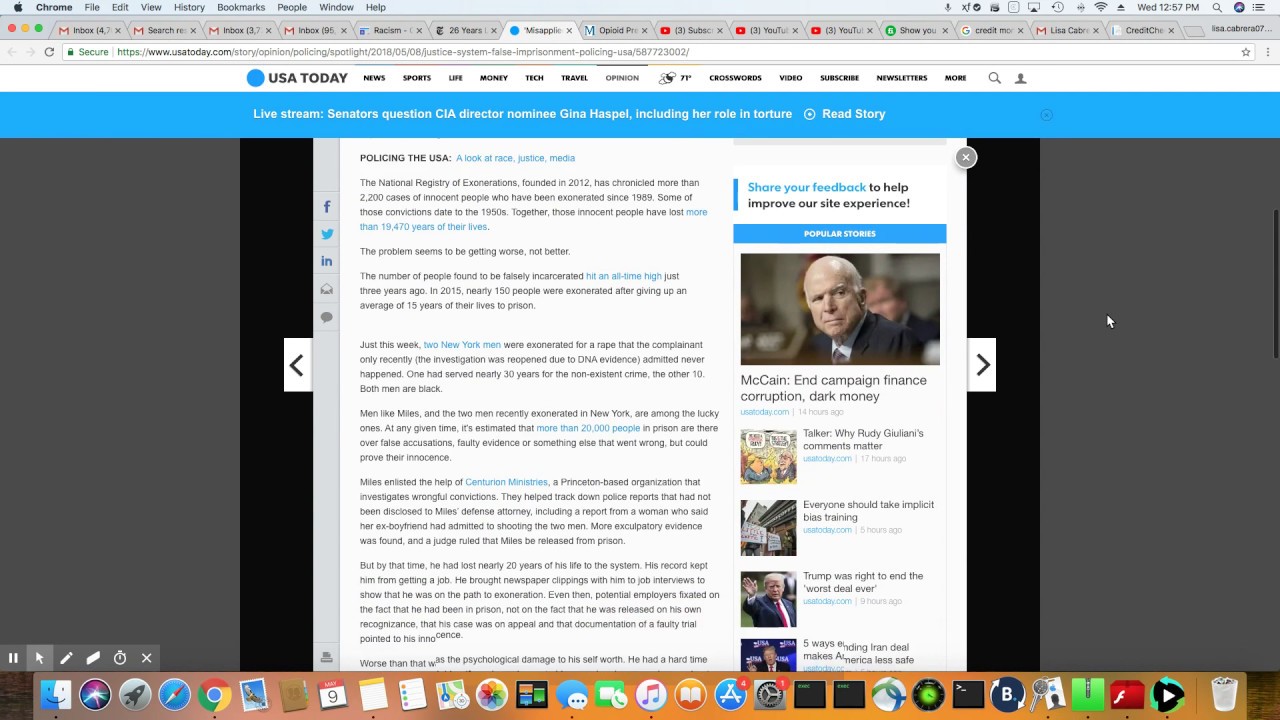**Detailed Caption for Screenshot Image:**

This image is a detailed screenshot of an entire computer desktop, specifically from a Mac. The top bar displays the Apple logo followed by the application in use, which is Chrome. The menu options available on the left side include: File, Edit, View, History, Bookmarks, People, Window, and Help, all in black text. On the right side, there is a series of icons indicating various system statuses, including Wi-Fi, microphone, and other utilities.

Below the top bar, the browser reveals multiple tabs open, approximately a couple of dozen. Among these are several Gmail tabs, articles from the New York Times, content related to racism and opioids, and multiple YouTube tabs. There are also tabs for credit check sites, and various other topics. The currently active tab is open to a USA Today article titled "Live Stream: Senators Question CIA Director Nominee Gina Haspel on Torture."

At the bottom of the desktop, the dock displays a range of application icons typical of a Mac environment. Visible icons include iTunes, Safari, Mail, and several others, confirming the use of macOS.

This detailed caption captures the extensive multi-tab browsing activity and desktop organization of the computer user.